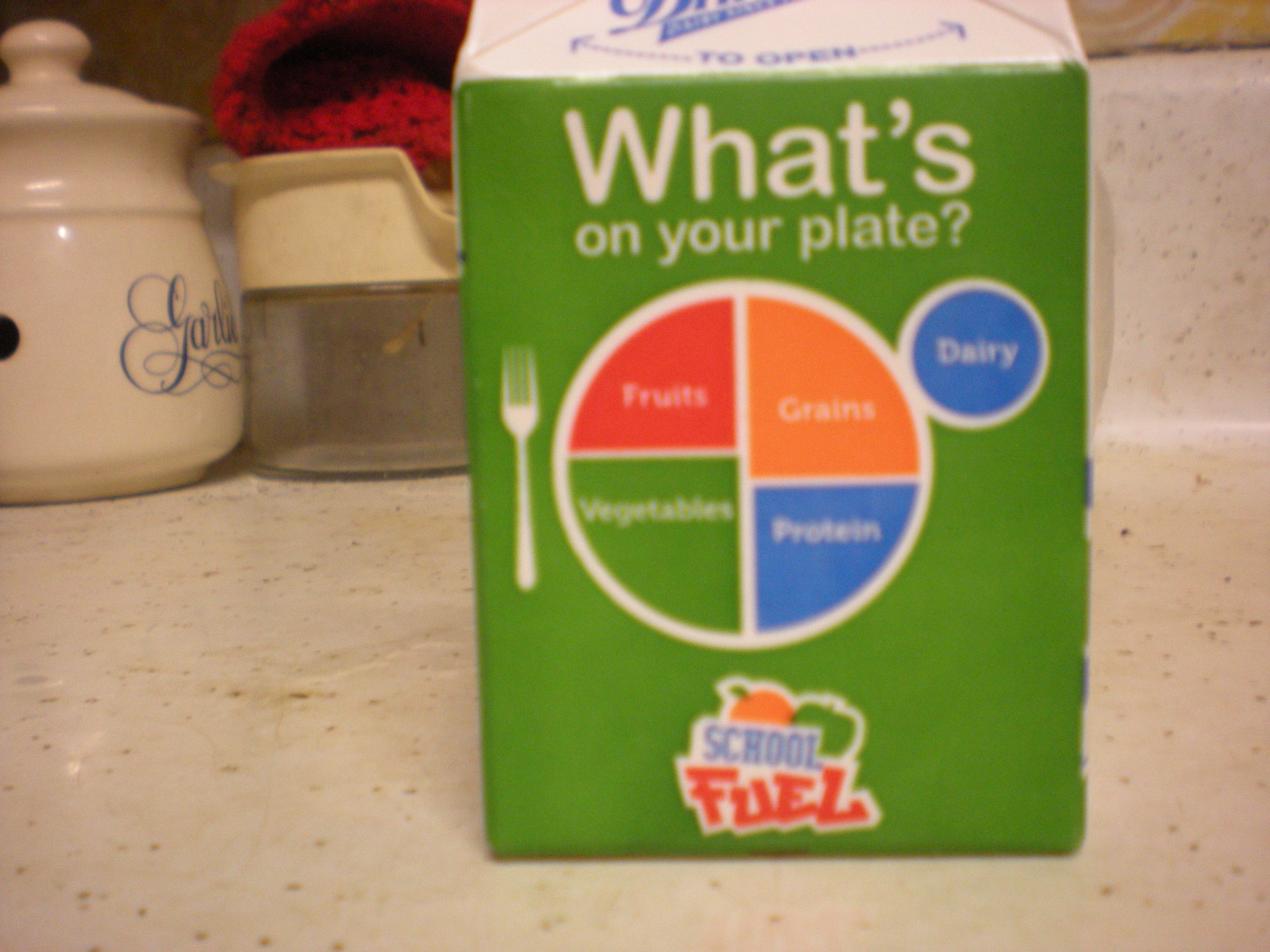This image features a high-resolution, close-up photograph of a small carton box positioned on a white granite kitchen countertop. The granite countertop is speckled with brown, black, and gold flecks, and part of the backsplash is visible in the background, complementing the countertop's appearance.

The focal point of the image is the small carton box, resembling a personal-sized juice or milk carton. The side facing the camera is green with white text at the top that reads "What's on your plate." Below this text is a circular pie chart divided into four sections: red labeled "Fruits," orange labeled "Grains," blue labeled "Protein," and green labeled "Vegetables," all in white text. Attached to this pie chart is a smaller blue circle labeled "Dairy." Additionally, a fork symbol is visible on the left side of the pie chart.

Underneath the pie chart, there is a logo featuring a school design with the words "School Fuel" in blue and red. The logo includes illustrations of an orange and an apple.

In the background, slightly to the left, there is a porcelain canister that possibly holds cookies or other items, with cursive text that appears to say "Garlic." Nearby, there is a small plastic container, and a red knitted cloth is draped over it. These elements add a domestic touch to the kitchen setting, enhancing the overall ambiance of the image.